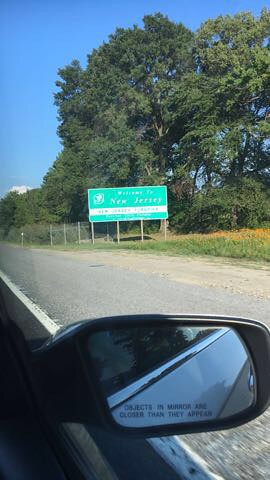This photograph, taken from the passenger side of a moving car, captures a bright summer day on a highway. The lower portion of the image prominently features the car's side mirror, which bears the inscription, "Objects in mirror are closer than they appear." Ahead, the road shoulder is partially visible, with a goldenrod plant on the right side, and the gravel leading up to a lane marker. At the top half of the image, a cloudless, light blue sky dominates, except for a portion of white clouds on the middle left, peeking above a tree line. The trees, full and lush with dark green leaves, extend horizontally across the middle of the image. In front of the trees stands a large green sign that reads "Welcome to New Jersey" in white writing, featuring a horizontal white line across it. The sign is mounted on four posts, with a chain-link fence visible behind it. The overall scene is a picturesque capture of a road trip in New Jersey on a clear, sunny day.